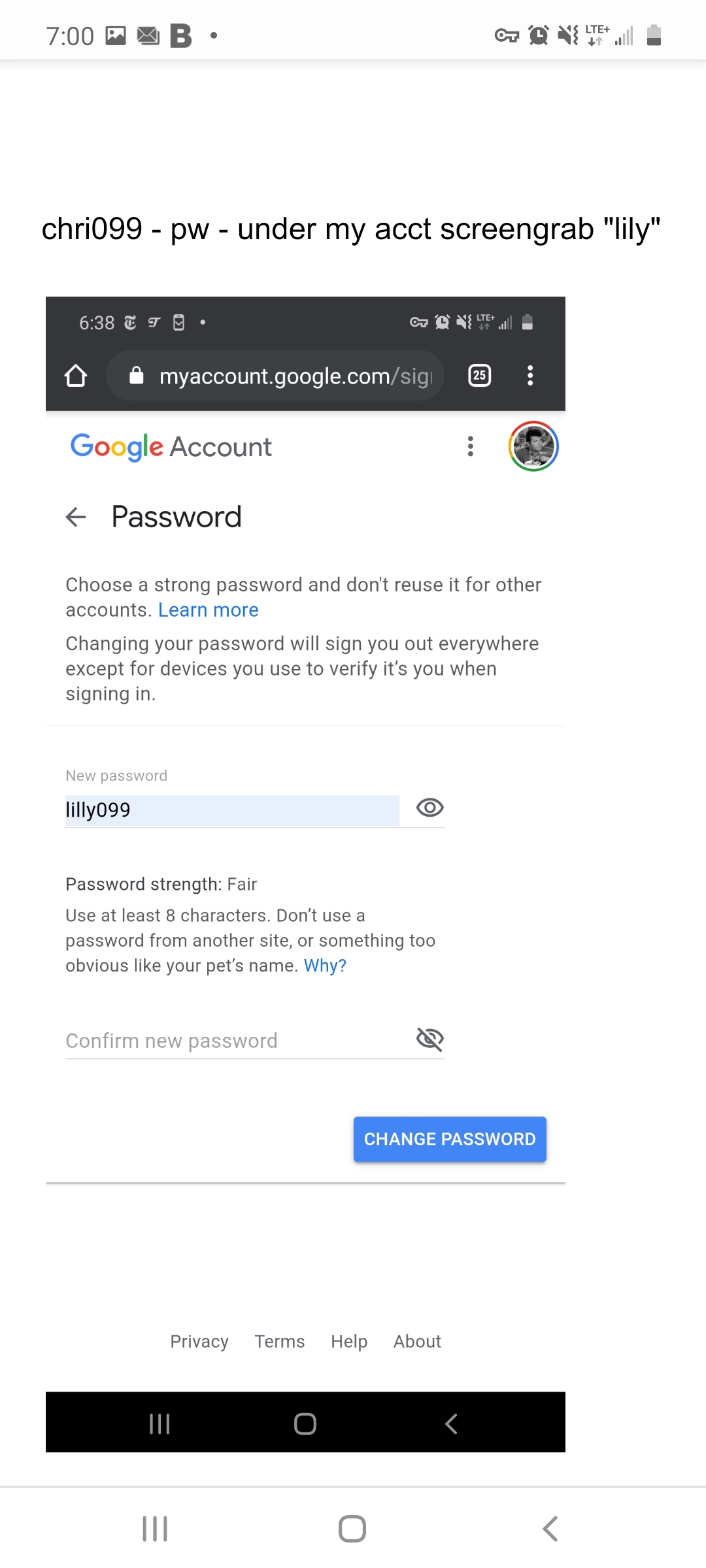The image appears to be a screenshot of a mobile phone screen captured at 7:00 AM. The screen displays a Google account password change page. At the top, under the user's account details, there is a string "CHRI 099 - PW - green" and the user's name, "Lily." The page instructs the user to choose a strong password and not to reuse it for other accounts. There's a hyperlink labeled "Learn more" that offers additional information. It also notes that changing the password will sign the user out of all devices except those used to verify their identity during sign-in. A new password, "Lily099," has been entered, with the password strength rated as "fair." Instructions advise using at least eight characters and not using passwords from other sites or obvious choices like pet names.